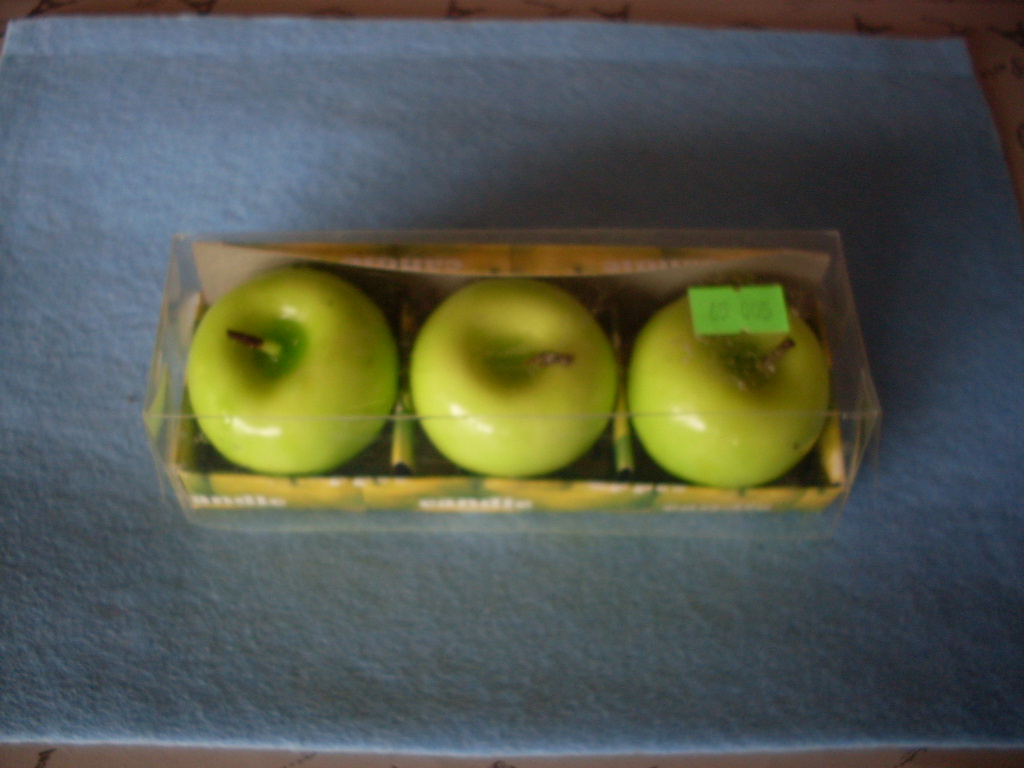The image depicts a slightly blurry close-up of three green apples, which are actually candles designed to look like apples. Each "apple" candle has a brown stem that resembles a wick. The candles are neatly arranged in a divided, brown cardboard carton that sits under a clear, rectangular plastic cover. There is a green price sticker in the upper right corner of the container, though the exact price is difficult to discern. The candles and carton rest on a blue cloth or towel, with a brown table or marble counter seen around the edges of the cloth. Additionally, the front of the carton features white writing, likely indicating that these are indeed candles, although the text is somewhat blurry and hard to read. The overall impression is of a neatly packaged and realistic-looking set of apple candles, carefully presented for sale or display.